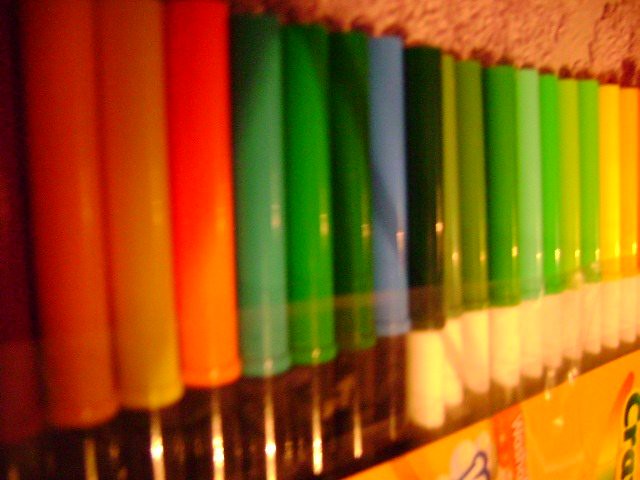A detailed close-up photograph of a pack of Crayola markers, still encased in their plastic packaging, reveals an array of colorful caps indicating the wide spectrum of hues inside. The markers, neatly aligned, protrude from a vibrant yellow and red package adorned with the Crayola logo in bold black lettering. The shades transition from warm oranges and yellows to a plethora of greens, including light green, grass green, dark green, very dark green, and other nuanced shades. Among the greens, there are also light blues, purplish-blues, and some markers with white and black bodies for grip. The background features a light beige rug along the top edge and possibly a pink blanket or carpet below, adding a cozy ambiance to the image, which appears to be taken with a personal camera, emphasizing the vibrant details up close.